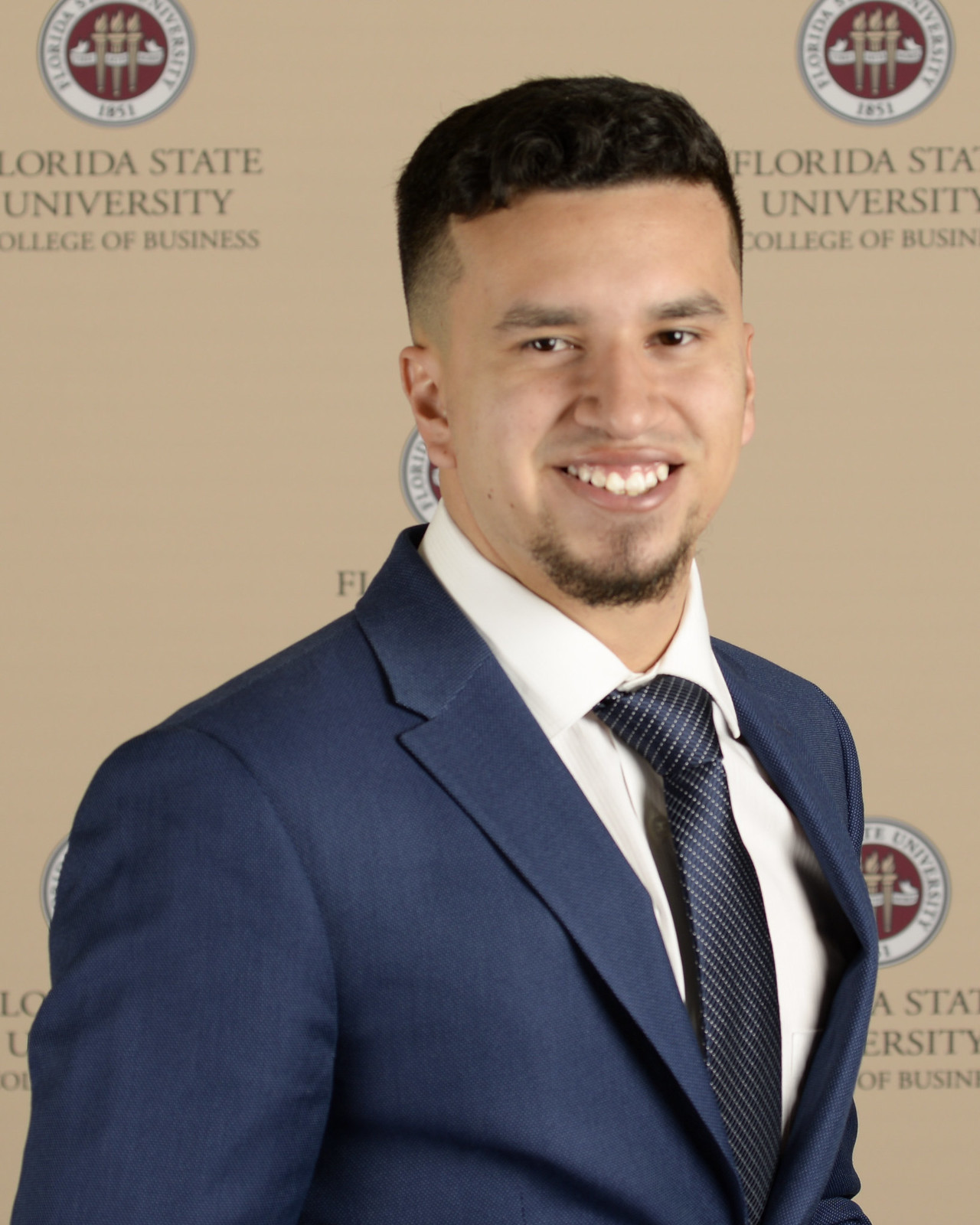The image features a young man in his early 20s, positioned against a tan-colored background adorned with multiple Florida State University College of Business logos. The most prominent logo is a round red emblem, outlined in white, displaying three gold-lit torches intertwined with a white banner. The text "Florida State University" and the founding year "1851" encircle the logo. The young man, with light brown skin, has short black hair styled in an undercut, with the sides of his head shaved nearly bald. He sports a beard on his chin, sans mustache. Dressed in a navy blue suit, a white shirt, and a blue tie with white polka dots, he faces the camera with a wide smile, revealing his top row of teeth. The rectangular photo captures him from the mid-torso up, standing confidently in the center of the frame, set against the repeated backdrop of the college's emblem.